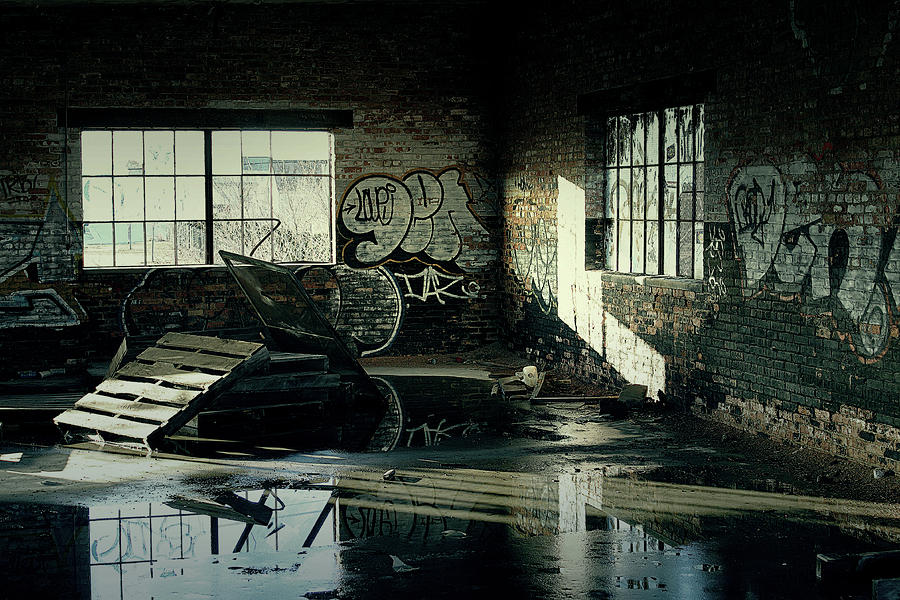This photograph captures the desolate interior of an abandoned warehouse or factory, where the signs of decay and disuse are evident. The focus is on a dimly-lit corner, intersected by two large windows that allow ambient daylight to seep through, casting a muted glow across the room. The windows, missing some panels, lend an air of dereliction and permit just enough light to highlight the room's grimy and wet conditions. The floor is speckled with puddles, indicating recent rain and possibly a compromised roof, creating reflections of the surrounding walls.

Both walls of the corner are adorned with vivid graffiti, primarily in white, but also featuring some black markings. The exposed brick and worn tiles add to the atmosphere of abandonment. Positioned within this damp space is a pallet, partially submerged in the standing water, alongside what appears to be a stacked screen door and other pieces of wood. The overall scene is one of neglect and urban decay, captured under the diffuse light of a cloudy daytime.